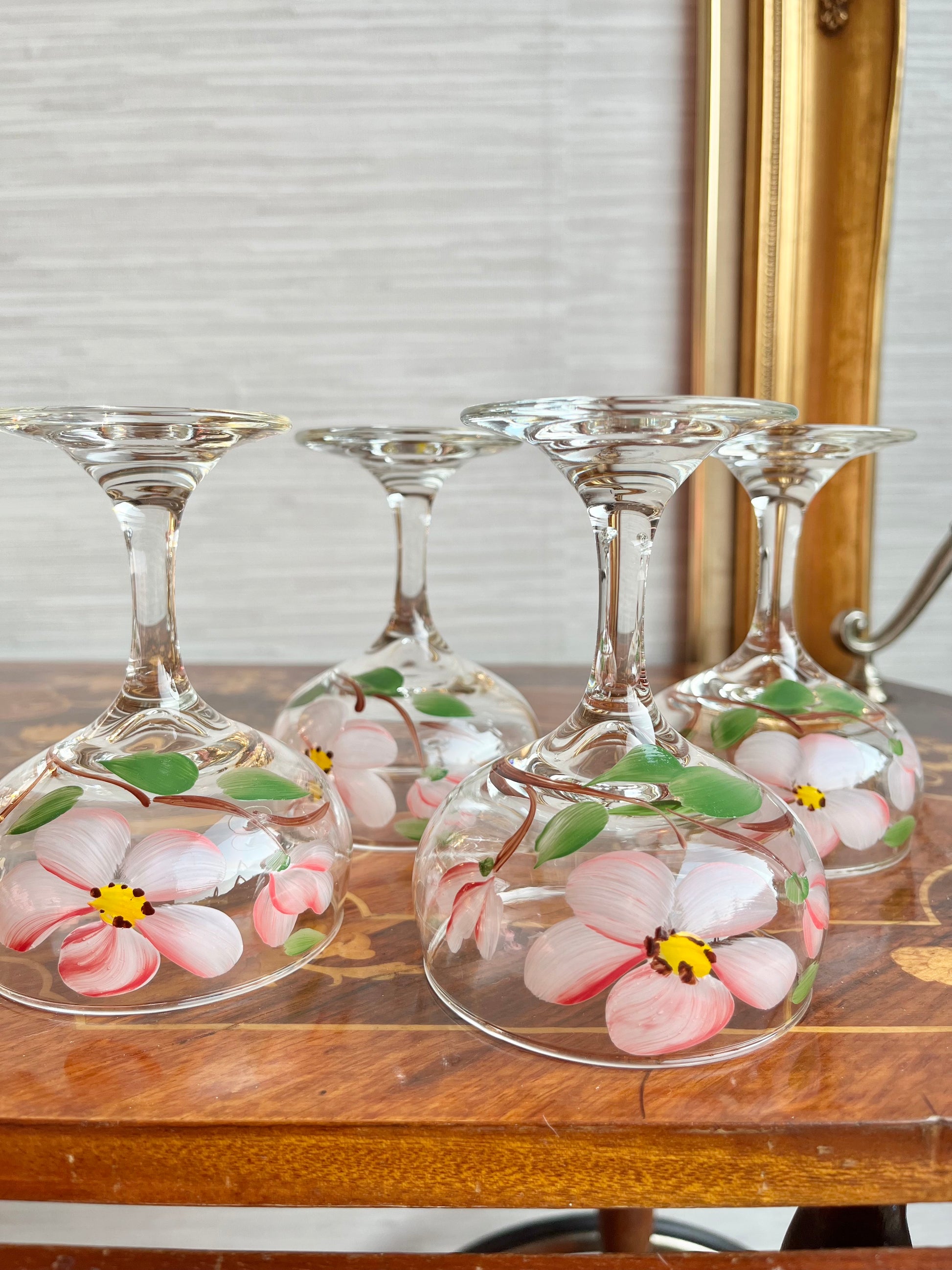This indoor photographic image showcases four upside-down wine glasses arranged delicately on a brown wooden table. Each glass is adorned with intricate floral patterns featuring pink flowers characterized by five petals with white edges, vibrant yellow centers, and subtle red dots around the center. The flowers are complemented by brown twigs and green leaves, creating a fresh and elegant look. In the background, a gray and white wall is visible, along with what appears to be a golden frame or wainscoting, adding a touch of sophistication to the setting. The overall aesthetic is characterized by a blend of natural floral beauty and refined interior decor.